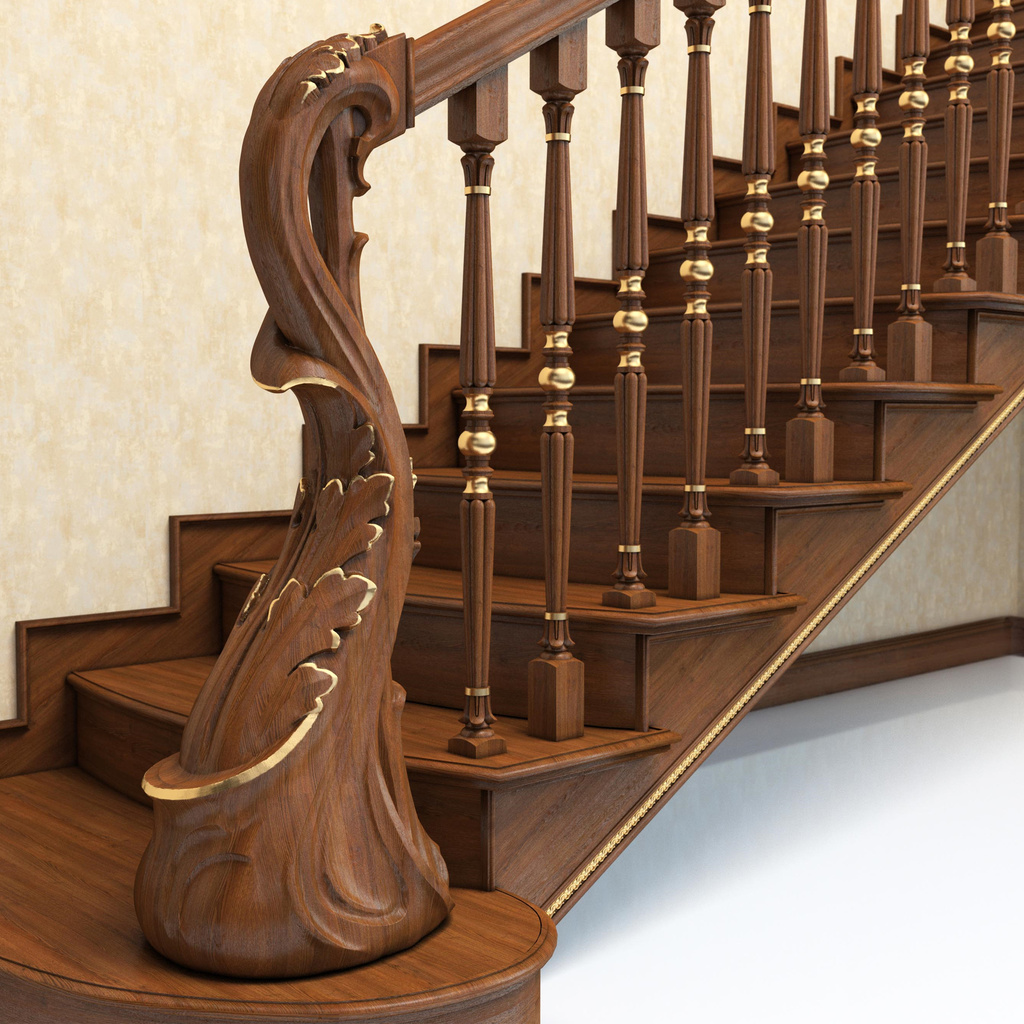This image captures a close-up of the lower half of a staircase, exquisitely designed with intricate details. The stairs themselves are made of a dark, polished brown wood, perhaps a hazelnut shade, leading upwards. Each step is accompanied by spindles that feature gold ball-shaped designs in their centers, adding a touch of elegance. The railing is of the same dark wood and is supported by these spindles, which are thin and intricately crafted. 

At the base of the staircase, the newel post stands out with its elaborate carvings, designed to resemble a tree trunk with branches and leaves, further adorned with gold accents that highlight the leaf-like patterns. The background features a beige, textured wall, adding to the homely or office-like vibe of the setting. The floor below is white, indicating that this is at the entrance or lower level of the building.